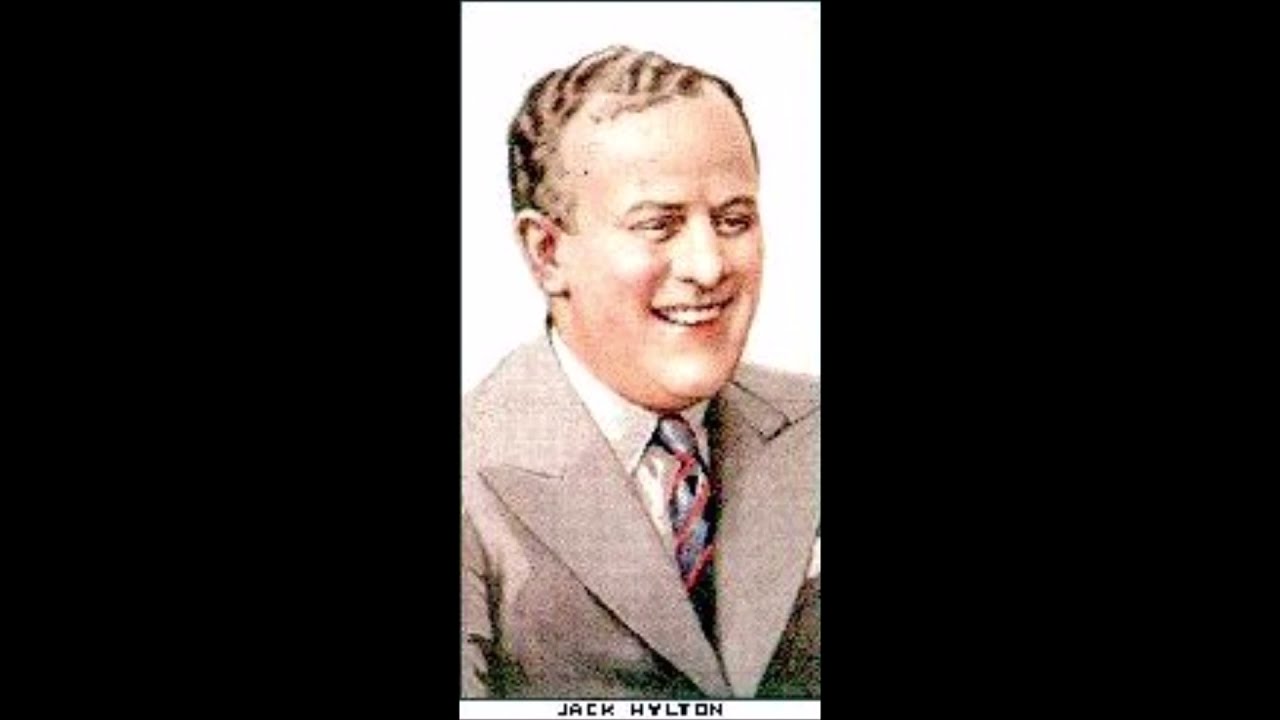The image is a poster divided into three vertical sections: the left and right thirds are completely black, while the central third features a detailed picture of a man on a white background. This central image appears to be either a drawing or a watercolor and has a grainy effect, giving it a vintage feel, possibly from the 1950s. The man, who is white, has short, curly brown hair, brown eyes, and expressive brown eyebrows. He is smiling slightly, with his mouth open just enough to reveal the top row of his teeth. He has a pointy, pudgy nose and is dressed in an old-style gray or tan suit. His outfit includes a white or gray button-up shirt and a blue tie with diagonal red stripes. He faces slightly to the right. At the bottom of this image, in all capital letters, the name "Jack Hylton" is prominently displayed.